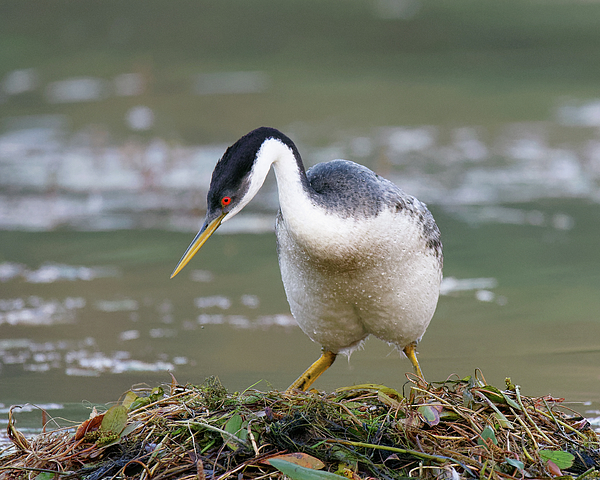This is a close-up, color photograph of a kingfisher standing on a nest-like mat of vegetation at the water's edge. The bird features a striking long curved neck with a dark blue strip running continuously from the top of its head down the back of its neck. Its beak is pointed and yellow with a hint of blue on top, and a notable red eye is visible on the left side of its head. The kingfisher's head, and the back of its neck are bordered by a gray stripe around the eye, continuing onto the adjacent part of the beak. The lower part of the bird, including its throat, neck, and belly, are pure white, while its back displays varying shades of dark and light gray. Tiny water droplets are scattered across its body, glistening in the light. The backdrop features a sparkling grayish-green water with white ripples, invoking a realistic beach area scene where sand and ocean waves meet.